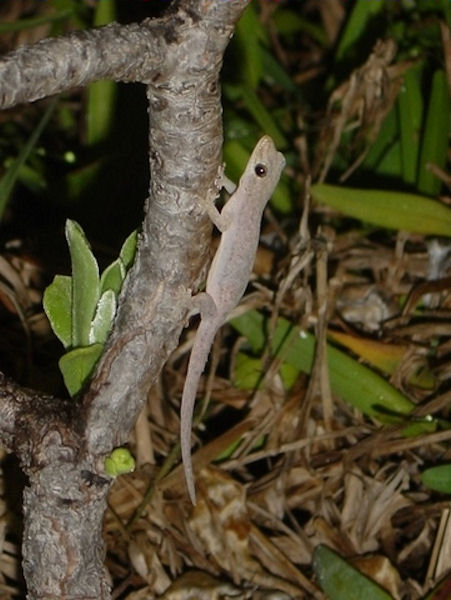In this captivating wildlife photograph, a brownish gecko clings vertically to a tree branch that occupies the left-hand side of the image. Positioned near the base of the tree, the gecko's tail points down while its nose faces upwards towards the top of the photo. Its back legs are splayed outward, and the front legs are bent as if performing push-ups, showcasing the unique adhesive ability of geckos. The gecko's glossy, beady black eye is turned towards the camera, giving an impression of vigilant stillness. The background reveals a forest floor covered in a mixture of brown leaf litter and large, glossy, tropical leaves, with some greenery sprouting from the forest carpet. Bathed in the nighttime illumination provided by the cameraman, a small nub of new growth is visible near the bottom of the living branch, adding a touch of vibrant green to the scene.